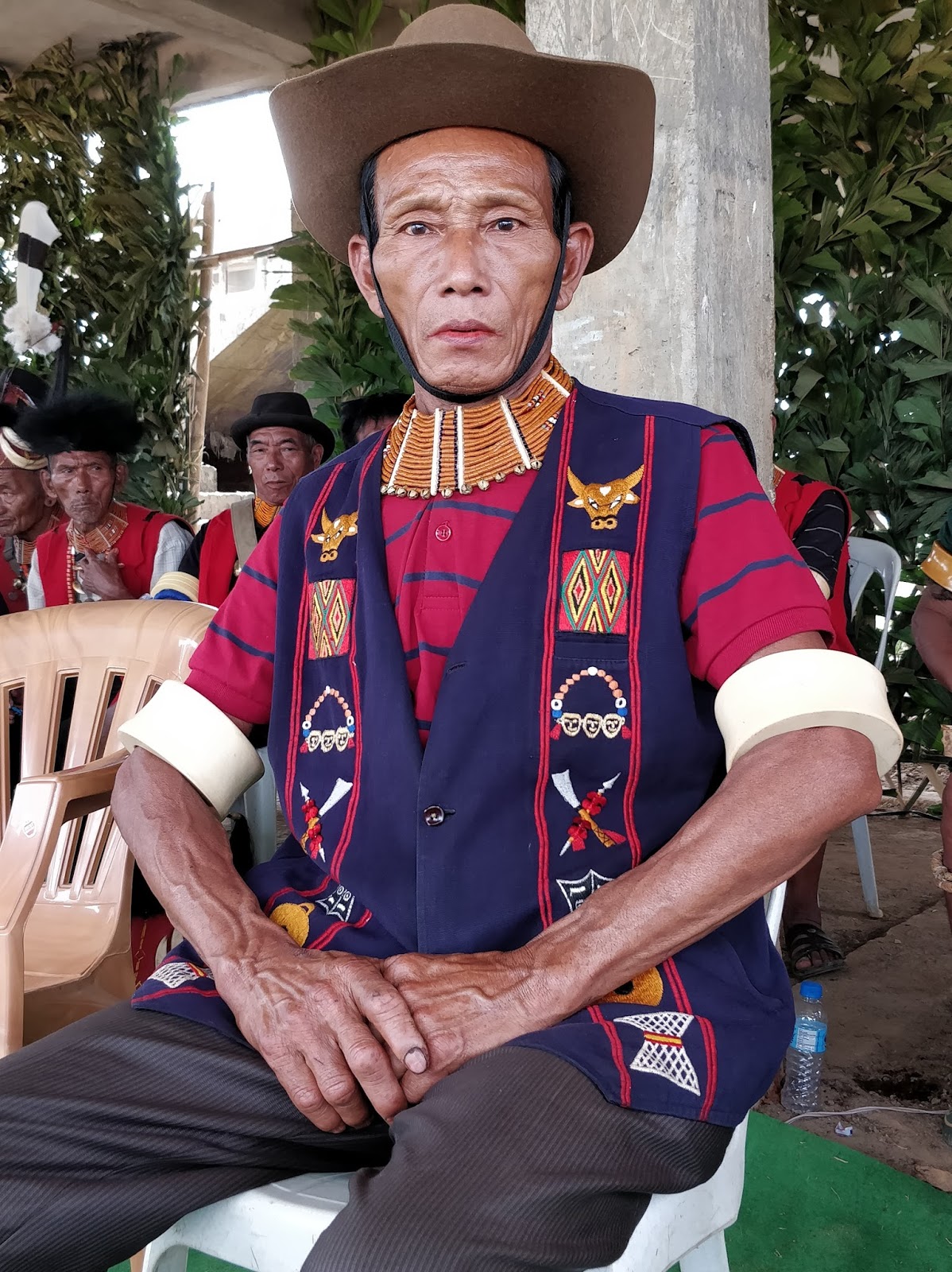In the image, an older man who appears to be of Native American descent is seated on a white plastic chair, positioned facing the camera. He wears a distinctive brown cowboy hat with a strap under his chin, which secures his black hair. His attire includes a short-sleeved red shirt adorned with thin blue horizontal stripes. Over this, he sports a navy vest featuring intricate tribal and cultural designs, including symmetrically placed patterns that resemble hunting scenes, masks, and possibly a spear. His dark brown dress pants complement his ensemble, and he has what seems like thick masking tapes above each elbow.

The man has a tanned complexion and no facial hair. His hands rest in his lap, fingers intertwined. In the background, the scene appears to be set in a porch area with a garden-like atmosphere, characterized by trees and grass. There are four other men visible off to his right; they too wear traditional attire with similar vests and a variety of headwear, including black fedoras and fuzzy hats. The setting and attire suggest a culturally significant context, with an emphasis on heritage and traditional clothing.